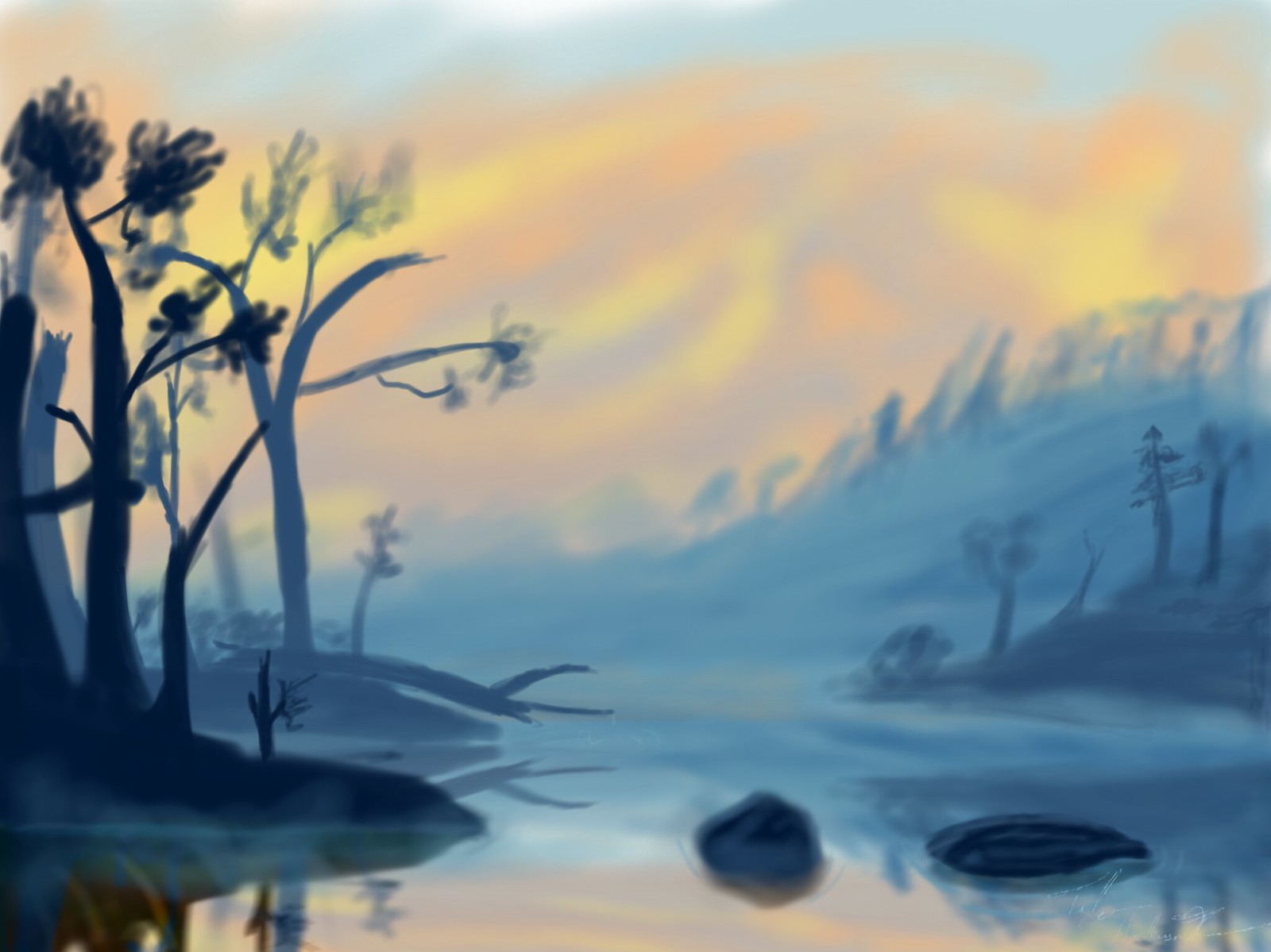This image appears to depict an intricate painted landscape. On the left side, tall, black trees with dense clusters of dark leaves stand prominently. To their right, a striking body of water starts with a white-pink hue at its base and features two prominent black rock-like formations. As the water extends into the background, it shifts to a vibrant blue, accented with streaks of dark blue.

On the right-hand side, a stretch of dark gray land is visible, dotted with small, vertically standing trees. In the distant background, there is a light blue, hill-like expanse marked with fine black lines, suggesting the presence of distant trees. Overhead, the sky is a mesmerizing blend of light purple, yellow, and orange hues, with a touch of light blue peeking through near the top, completing this captivating outdoor scene.